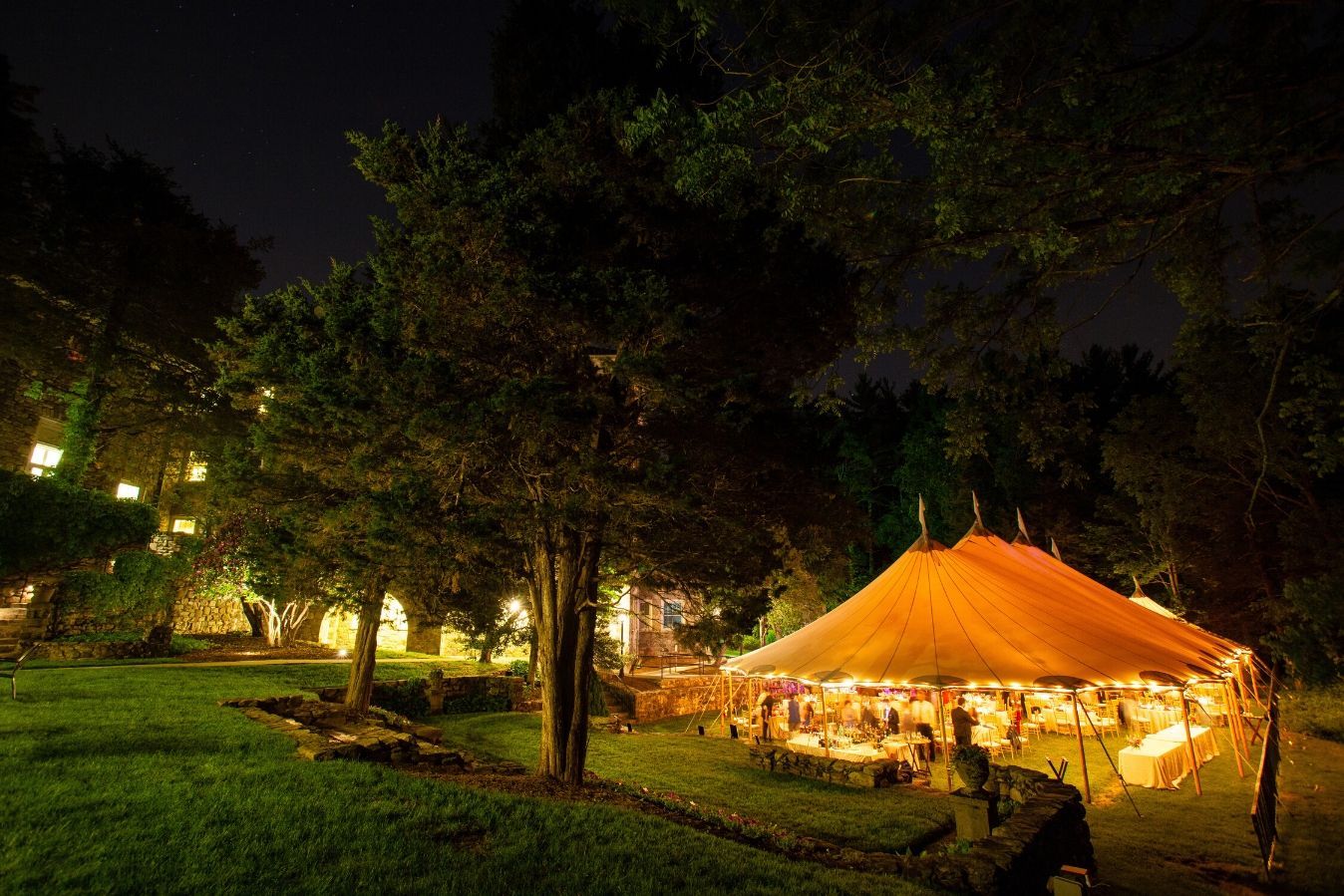This vivid color photograph captures a serene park scene at night, illuminated solely by ambient light. A carpet of lush green grass stretches across the ground, bordered by numerous tall, majestic trees that stand like silent sentinels in the night. In the background, a stately stone building glows warmly, its numerous windows radiating a soft, inviting light. Near the right edge of the image, a large, elegantly adorned tent stands open, revealing a formal event in progress. Inside the tent, long tables draped in pristine white tablecloths are arranged neatly, laden with an array of food and glasses. Guests move about gracefully, engaging in conversation under the gently glowing lights. The sky overhead is a deep, velvety black, adding a tranquil backdrop to the lively scene below. This well-composed photograph captures the essence of a sophisticated evening gathering, shrouded in the calm of nature's embrace.